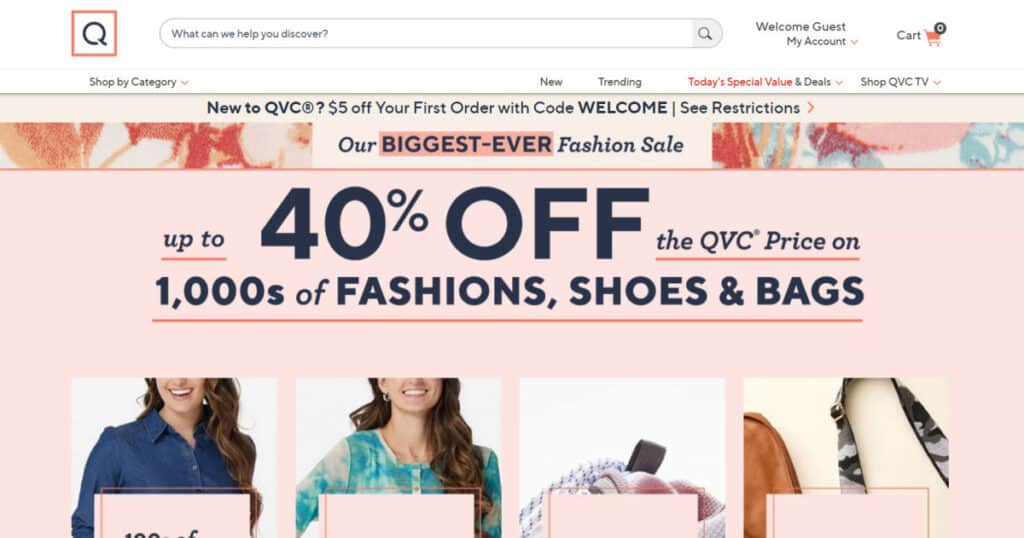This screenshot captures the landing page of the online retailer QVC. At the top, there is a prominent search bar, flanked on the left by the QVC icon. To the right of the search bar, the user interface welcomes guests and includes sections for "My Account" and a shopping cart icon at the far right. 

Below this top header, a large banner announces, "New to QVC? $5 off your first order with code WELCOME. See restrictions." Directly below this banner, there’s another message in large, bold text proclaiming, "Our Biggest Ever Fashion Sale," with "Biggest Ever" highlighted in pink for emphasis. The sale offers up to 40% off on thousands of fashions, shoes, and bags.

The main body of the page is divided into four sections, each featuring different images that presumably correspond to various categories or promotional offers within the sale. This meticulously organized layout underscores QVC's extensive and enticing promotional campaign.

In summary, this is a detailed look at QVC's landing page, showcasing a significant promotional offer aimed at attracting customers, particularly new ones, with visually striking banners and highlighted text to draw attention to their biggest fashion sale yet.